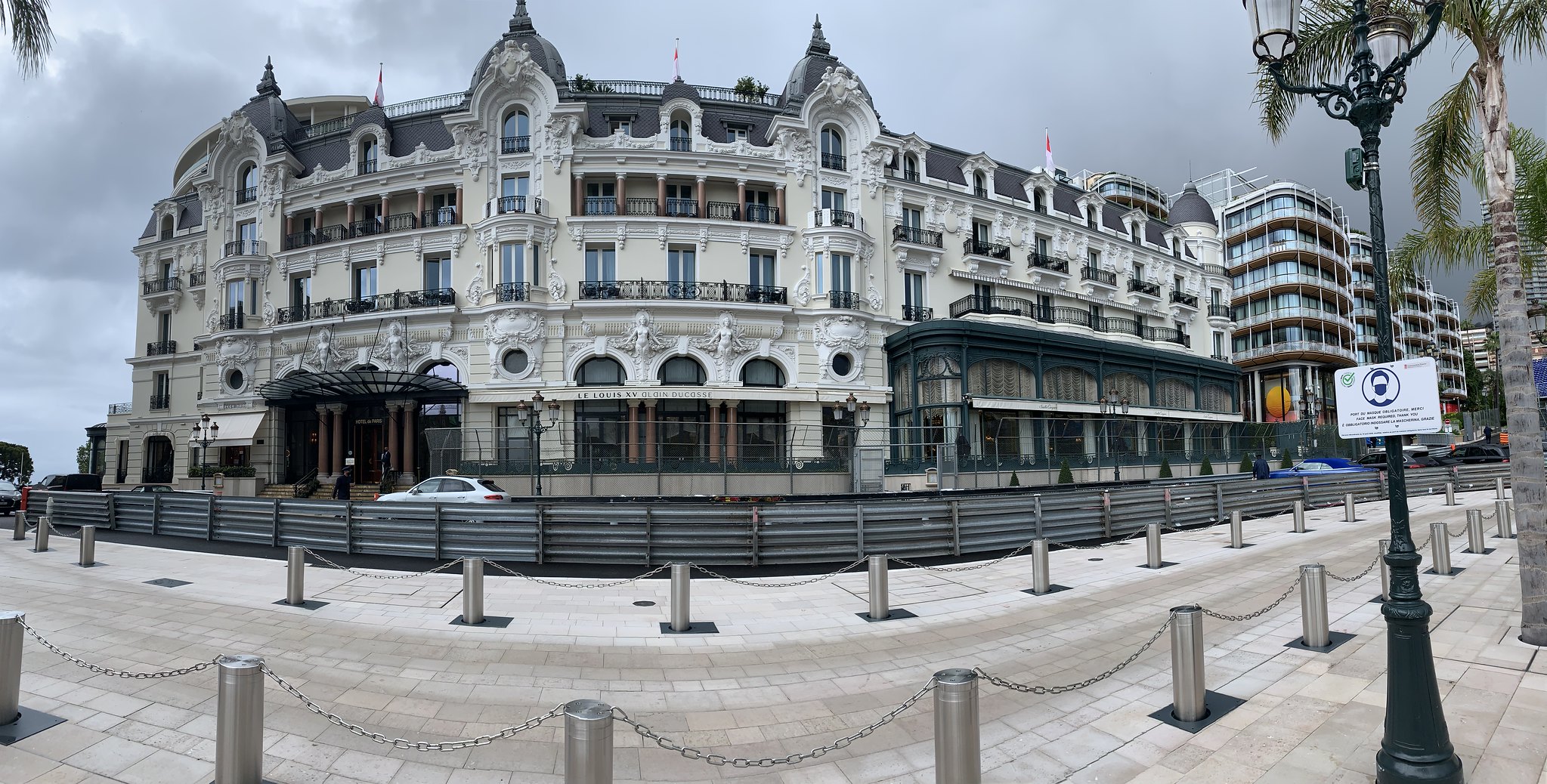The panoramic photograph captures a grand, classical-style building that could be situated in Monte Carlo, suggested by the familiar Formula One race barriers lining the road in front. The structure, predominantly white with decorative gray roof, black balconies, and numerous arches and windows, showcases historical elegance. The building is adorned with flags at the top, and the surrounding environment is meticulously clean, with no people visible, suggesting either early morning or preparation for an event. The sky above is moody and clouded, exuding a wintry autumn atmosphere with thick clouds masking the blue sky. In the foreground, the street is paved with white stones and lined with metal cylinders and chains. Positioned in front of the building and partly obscured by the barriers, a silver car drives by, with palm trees flanking the scene on the right. On the far left, there is a black pickup truck and some modern buildings in the background, adding contrast to the scene. A stylish lamppost with triple lights and a sign displaying an icon of a person with a black face mask completes the sophisticated yet serene scene.